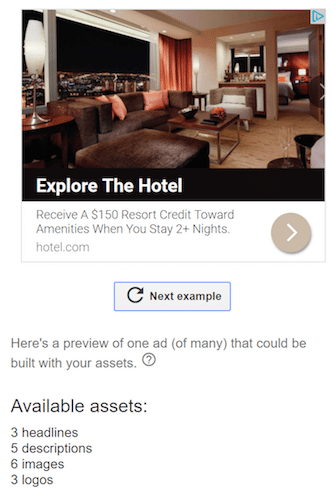The image showcases a high-class hotel room with a stunning view through its large window. The room appears to be fully furnished, featuring what seems to be a kitchen or at least a kitchen area, alongside a visible bedroom. This image is part of a smartphone website under the page titled "Explore the Hotel."

Beneath the image is a promotional banner reading, "Receive a $150 resort credit toward amenities when you stay two plus nights," followed by the website's name, hotel.com. There is also an interactive element: a tan circle with a white-facing arrow.

Further down, there's a gray box bordered in purple with an option to refresh, labeled "Next Example." Accompanying this section is a brief explanation: "Here's a preview of one ad (of many) that can be built with your assets." Additionally, a circular icon with a question mark provides information that available assets in descending order include three headlines, five descriptions, six images, and three logos.